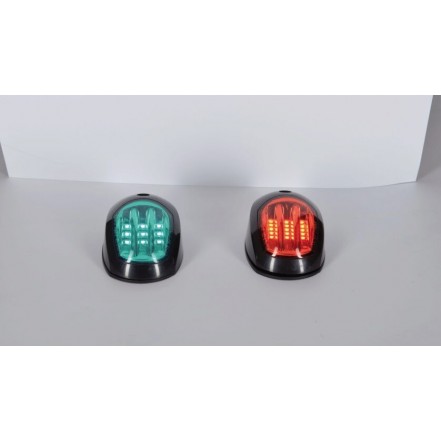The image depicts two identical black plastic devices sitting side-by-side on a white table, with a standing white piece of paper or poster board visible in the upper third of the photograph. These devices, which have a shiny finish and are shaped similarly to computer mice, sport small black buttons centrally located on their tops. They each have oval-shaped clear sections near the back that emit light—one glows a pale greenish turquoise color while the other shines a red-orange hue. The background setup suggests a product photo arrangement typically used for online listings.